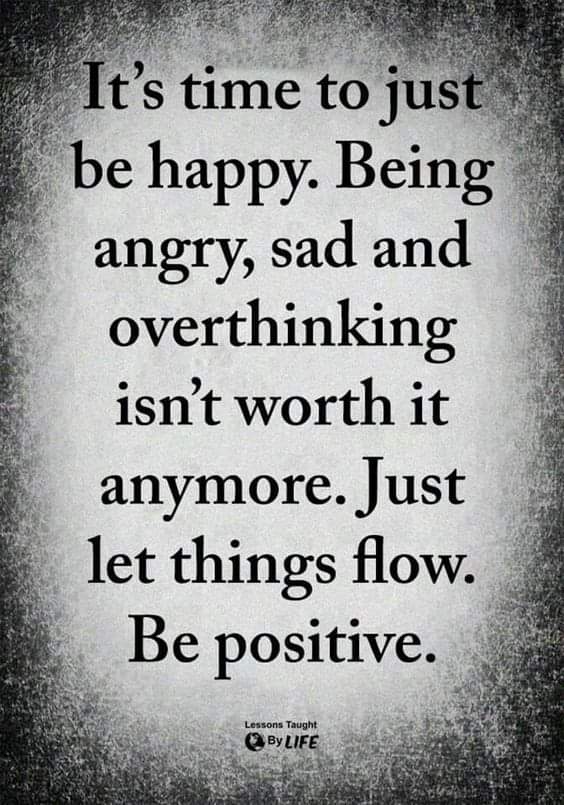This black and white poster features a powerful quote from Lessons Taught by Life. The backdrop has a gradated gray design that starts lighter in the center and transitions to a darker, more grungy texture at the edges, although the text remains unaffected by the grunge. The message is displayed in large, prominent text covering the entire image, reading: "It's time to just be happy. Being angry, sad, and overthinking isn't worth it anymore. Just let things flow. Be positive." At the bottom of the poster, in much smaller text, it says "Lessons Taught by Life," next to a small globe icon that symbolizes the word "Life." The simple yet profound message encourages positivity and the release of negative emotions.